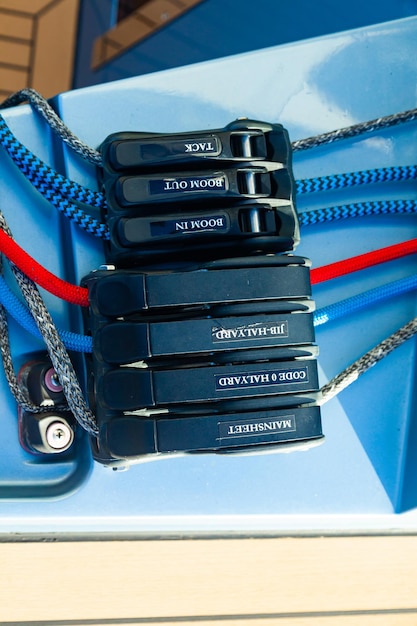The photograph showcases a black metal structure featuring various latches, each labeled with all-caps white writing, indicating their specific functions. Prominent labels include "MAIN SHEET," "CODE HALYARD," "JIB-HALYARD," "TACK," "BOOM OUT," and "BOOM IN." The latches appear to be horizontally aligned and are secured to a blue and white surface, suggesting they are part of a sailing ship's rigging system. Multiple climbing ropes, featuring distinct colors and patterns such as solid blue, red, white with black speckles, and blue with black zigzags, are threaded through these latches. The detailed labeling and the presence of various types of specialized ropes imply the setup is used for precise sailing maneuvers.